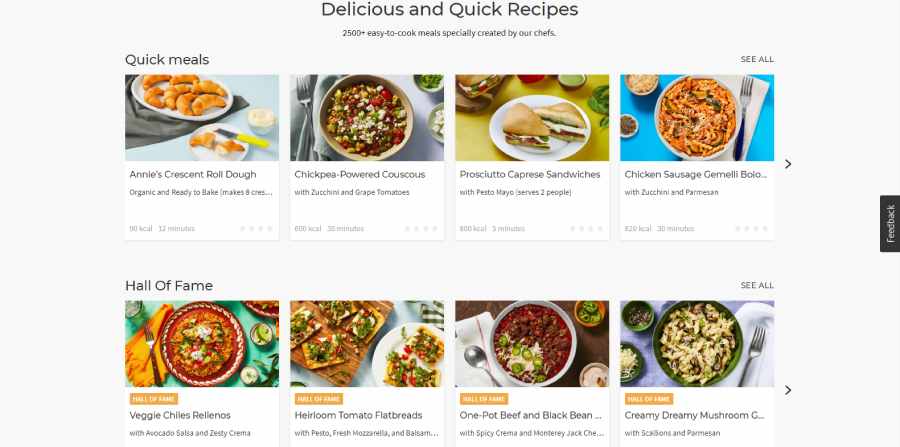**Screenshot of a Culinary Website**

The background of the website is an off-white color, giving it a clean and modern look. At the top, in black font, it reads: "Delicious and Quick Recipes: 2,500+ Easy-to-Cook Meals Specifically Created by Our Chefs."

Below this header, there are two rows of icons displaying different recipes, complete with enticing pictures of the finished dishes.

The first row is labeled "Quick Meals" in black font. It includes:
1. A photo of croissants labeled "Annie's Crescent Roll Dough - Organic and Ready to Bake."
2. A bowl of couscous accompanied by the text "Chickpea Powered Couscous with Zucchini and Grape Tomatoes."
3. A white plate with a cut-up sandwich, labeled "Prosciutto Caprese Sandwiches with Pesto Mayo - Serves Two People."
4. A bowl of pasta, labeled "Chicken Sausage Gemelli with Zucchini and Parmesan."

The row below is labeled "Hall of Fame" and features:
1. "Veggie Chiles Rellenos."
2. "Heirloom Tomato Flatbread."
3. "One-Pot Beef and Black Bean."
4. An image with the caption cut off, reading "Creamy Dreamy Mushroom Something." 

This detailed breakdown provides a comprehensive look at the various recipes showcased on the website, catering to users seeking both quick meals and all-time favorite dishes.